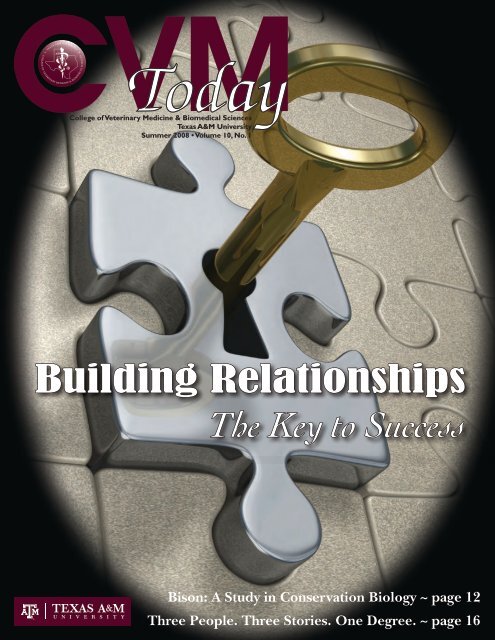The cover of what appears to be a textbook or a magazine for Texas A&M University prominently features the title "CVM Today" at the top, with "CVM" in maroon text and "Today" in white text. The main image displays a set of puzzle pieces with one raised piece that is metallic and contains a keyhole with a golden key inside. Beneath the image, the text reads "Building Relationships, The Key to Success" in white letters. Further down, additional text states "Bison: A Study in Conservation Biology" with a reference to page 12, and "Three People, Three Stories, One Degree" with a reference to page 16. The Texas A&M University logo is situated at the bottom left of the cover, indicating that this publication could be part of a student introduction packet or a similar informational resource.